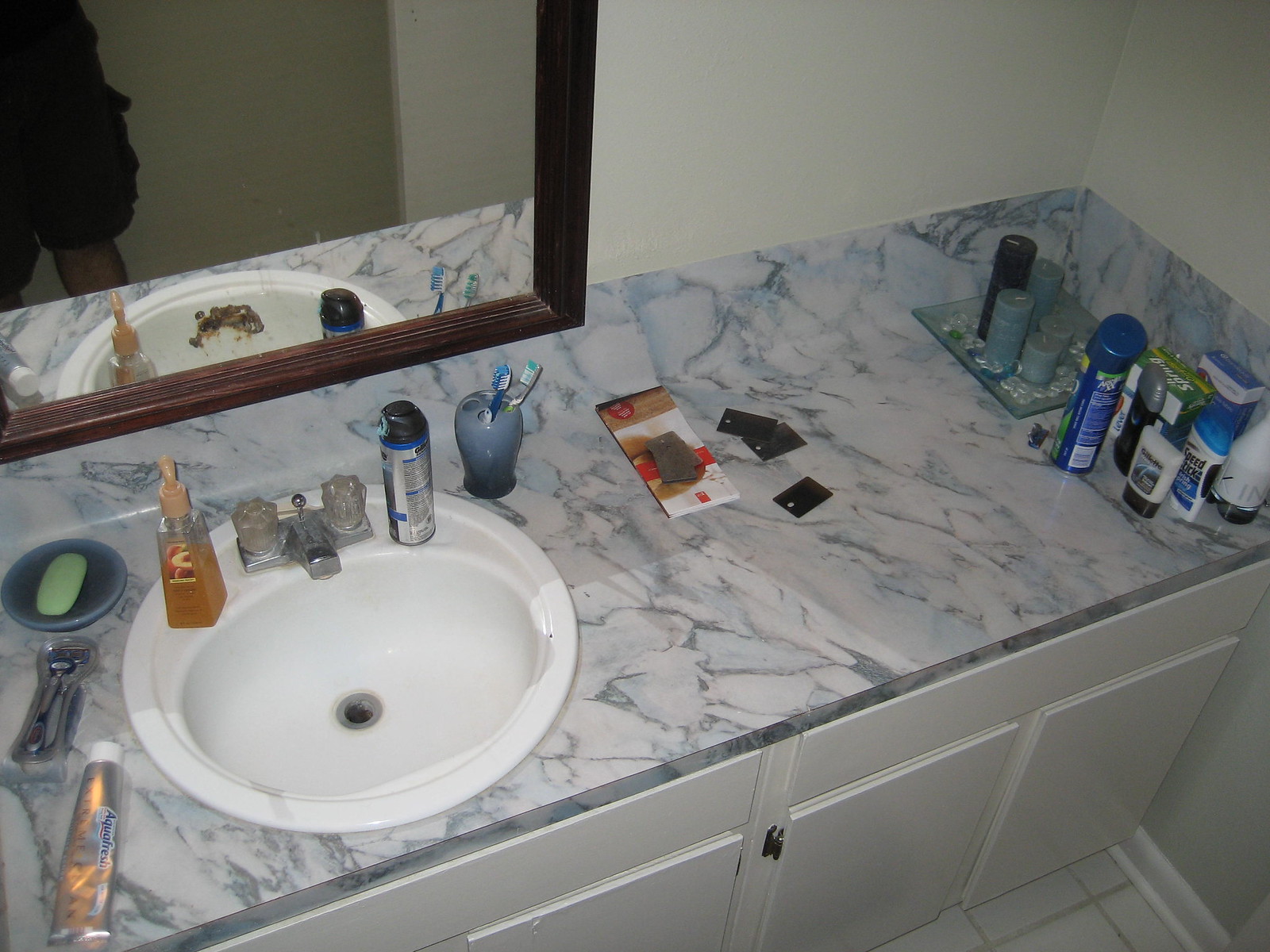The image presents a highly detailed, photorealistic depiction of a bathroom countertop made of gray and white granite. The countertop is methodically organized, with a white sink centrally positioned. The sink, circular in shape, is surrounded by white cabinetry featuring two open door handles at the bottom right, suggesting functional storage space.

On the right side of the countertop, there's an array of bathroom essentials neatly arranged. This collection includes various deodorants, soaps, hairsprays, and shaving creams. Above this array, a decorative plate holds an assortment of candles in black and blue shades, featuring varying sizes: two small, two medium, and one large black candle.

To the left of this setup are several cards or rectangular items, whose exact nature is unclear. Next to these, a blue, globe-shaped toothbrush holder contains multiple toothbrushes.

On the left side of the sink, additional personal care items are displayed. Here, another shaving cream stands beside a brown hand soap dispenser. Further to the left, more soap and an additional shaving cream tube are visible, accompanied by toothpaste, all contributing to the well-equipped and thoughtfully organized setup.